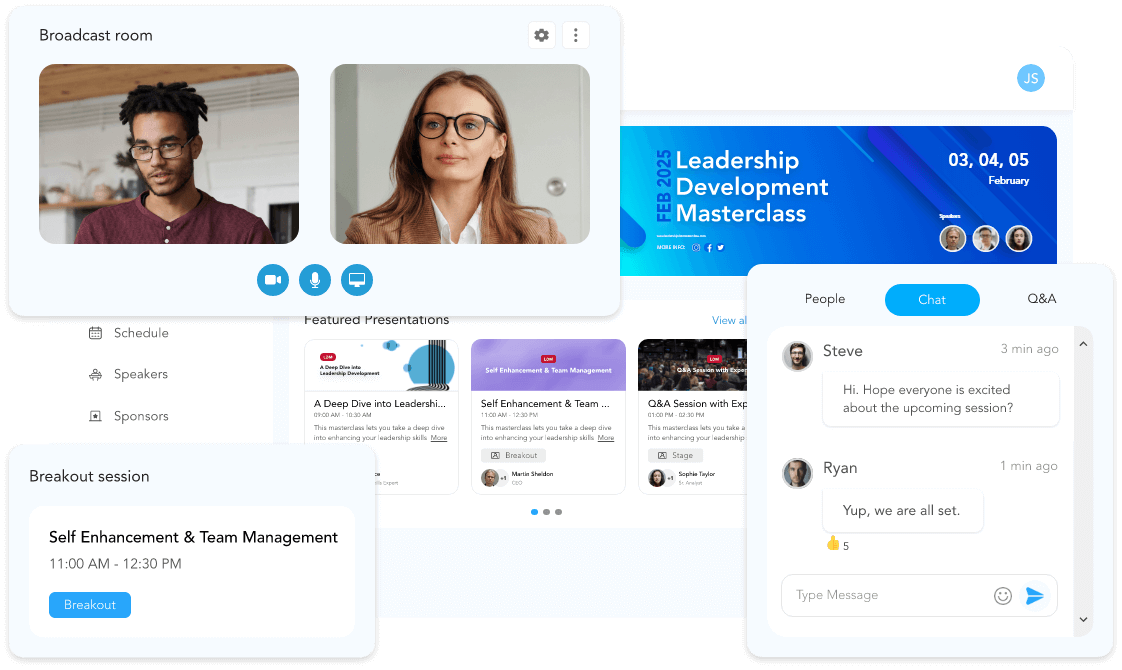The image portrays a dynamic screen with four overlapping windows, each displaying distinct elements. At the furthest back is the "Leadership Development Masterclass" website, which is an event scheduled for February 2025. This primary window highlights the key features of the masterclass, including topics such as "A Deep Dive into Leadership," "Self-Enhancement and Team," and a "Q&A Session with Experts."

In the mid-ground, another window shows a Zoom call between two individuals. On the left is a young man with short dreadlocks, wearing a collarless shirt with white buttons. Opposite him, on the right, is a woman with long hair and blue eyes, dressed in glasses, a white shirt, and a tan-colored jacket.

The third window, partially overlaid on the others, is a chat group message thread featuring an exchange between Steve and Ryan. The conversation seems to be actively ongoing.

Finally, a smaller notification window in the foreground indicates an upcoming breakout session titled "Self-Enhancement and Team Management."